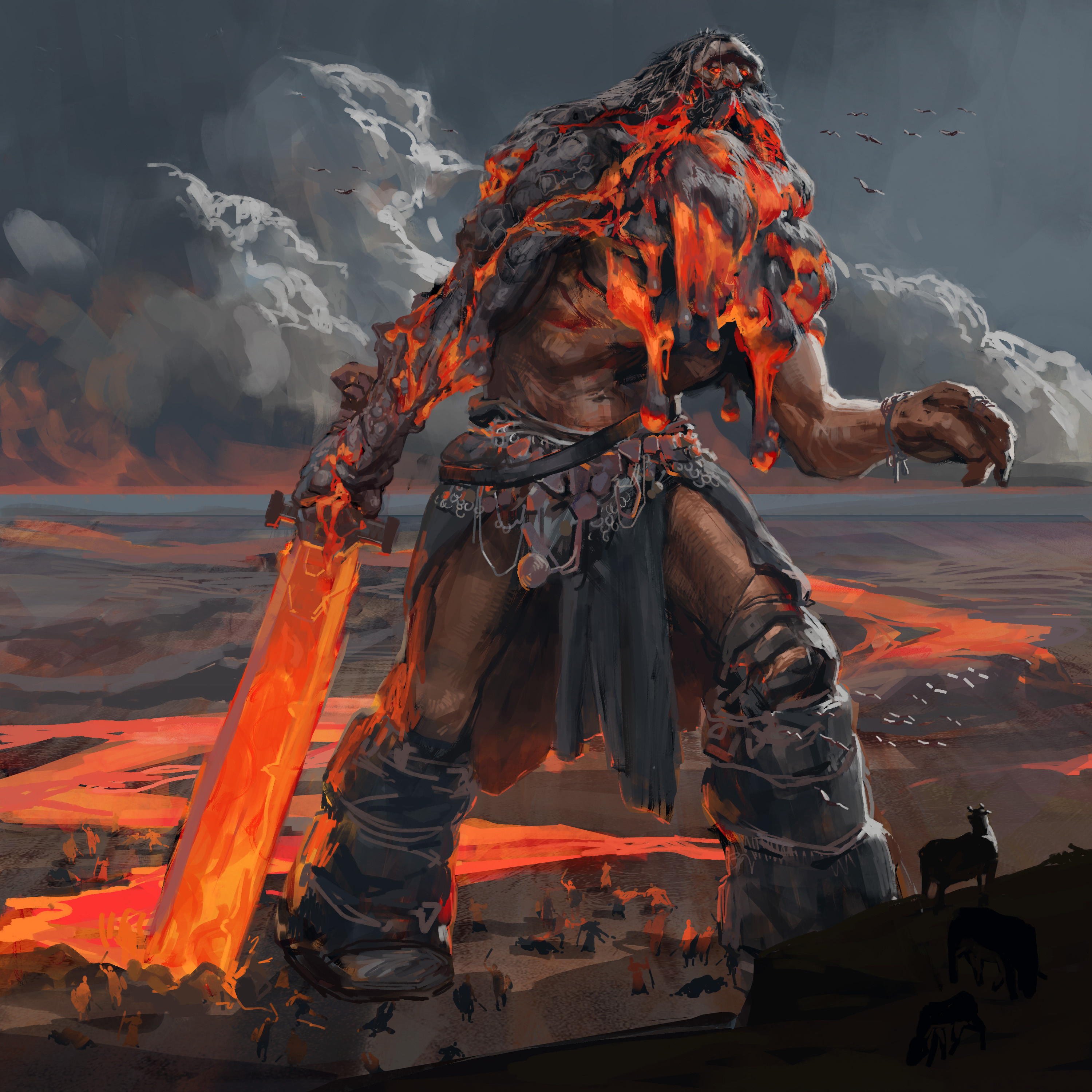In this detailed artist's painting, we observe a menacing titan standing amidst a haunting battlefield strewn with slain bodies. The medium appears to be watercolor, capturing a surreal and fantastical atmosphere. At the bottom of the image, the titan is prominently positioned among dark gray, lifeless forms on the ground, signifying a scene of recent destruction.

To the bottom right, the hillside hosts a small group of sheep or rams, with one creature turning its gaze towards the towering giant, adding a stark contrast between the tranquil animals and the chaos below.

The titan is clad in an elaborate fantasy attire reminiscent of Viking warriors. Its waist is encircled by a tattered skirt-like garment and a metallic belt adorned with various objects. The titan's lower limbs are wrapped in fur or leather, tightly bound with rope for a rugged look. In its right hand, it wields a mighty sword that appears to be forged from burning lava, glowing with intense yellow and orange hues. The sword’s base trails a winding river of lava that stretches into the distant desolate landscape.

The background reveals a deserted and barren terrain, almost lunar in its flatness. Dark clouds loom far off in the distance, casting an ominous shadow over the scene. While the sky is largely obscured, a hint of gray in the top-right corner reveals a flock of birds in flight, perhaps fleeing from the devastation below.

The titan’s head and beard are an extraordinary sight, composed of flowing, molten lava, which could imply that the creature is either the very source of the searing streams or engulfed by them. Its muscular physique is imposing, marked by thick, powerful thighs and a robust, well-defined torso.

Overall, this painting transports the viewer into a fantastical realm where titanic beings wage war in a desolate, apocalyptic landscape.